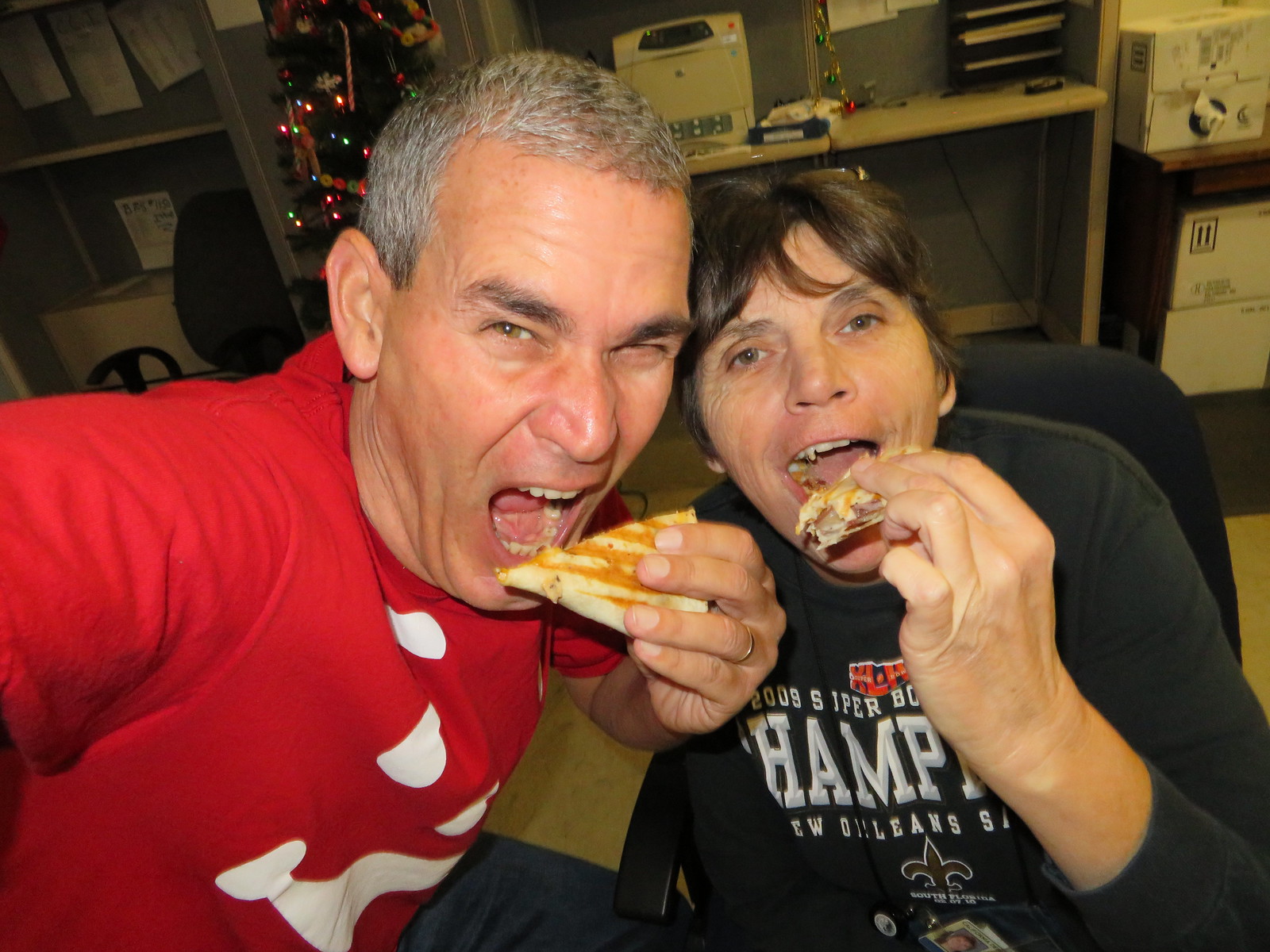Two people, a man and a woman, are taking a selfie in an office setting. The man on the left, with gray hair, is squinting one eye and has his mouth wide open, holding a triangular-shaped food item, possibly a slice of pizza or calzone, to his mouth. He wears a red shirt featuring a white face print. The woman on the right has brown hair and is also eating a similar triangular food item, taking a bite. She is seated in an office chair wearing a dark gray shirt with text reading "Champion, New Orleans Saints, 2009." Their expressions appear exaggerated as they pose for the camera, holding their food close to their mouths. The background features office equipment, cubicles, another office chair, and a small Christmas tree, indicating the photo was taken in an office environment.